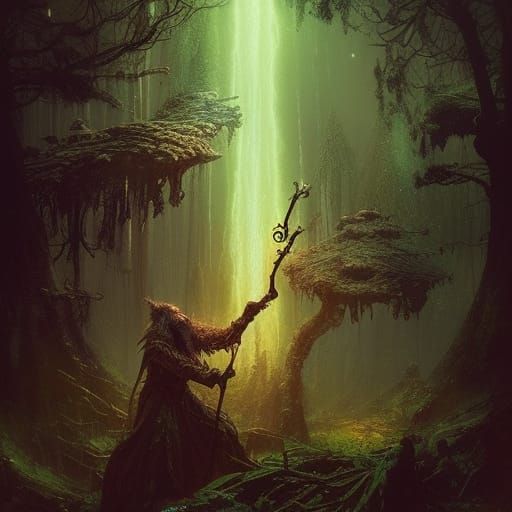The image depicts an eerie and surreal medieval forest scene characterized by lush foliage of greens and yellows, with trees bearing both eerie, black branches and willow-like leaves on either side. In the middle ground, the forest floor is strewn with grass and twigs, bathed in a green, mossy light filtered through the canopy. Dominating the foreground is a mysterious, human-like forest wizard made of moss and bark, clad in a long gown and a cap, and potentially sporting a beard. He holds a large, broken-off branch that serves as his staff, which he raises toward a tree as if casting a spell. Green light emanates from the center, contributing to the image's mystical atmosphere, as beams of light cut through the forest, creating a fairy-tale-like ambiance.